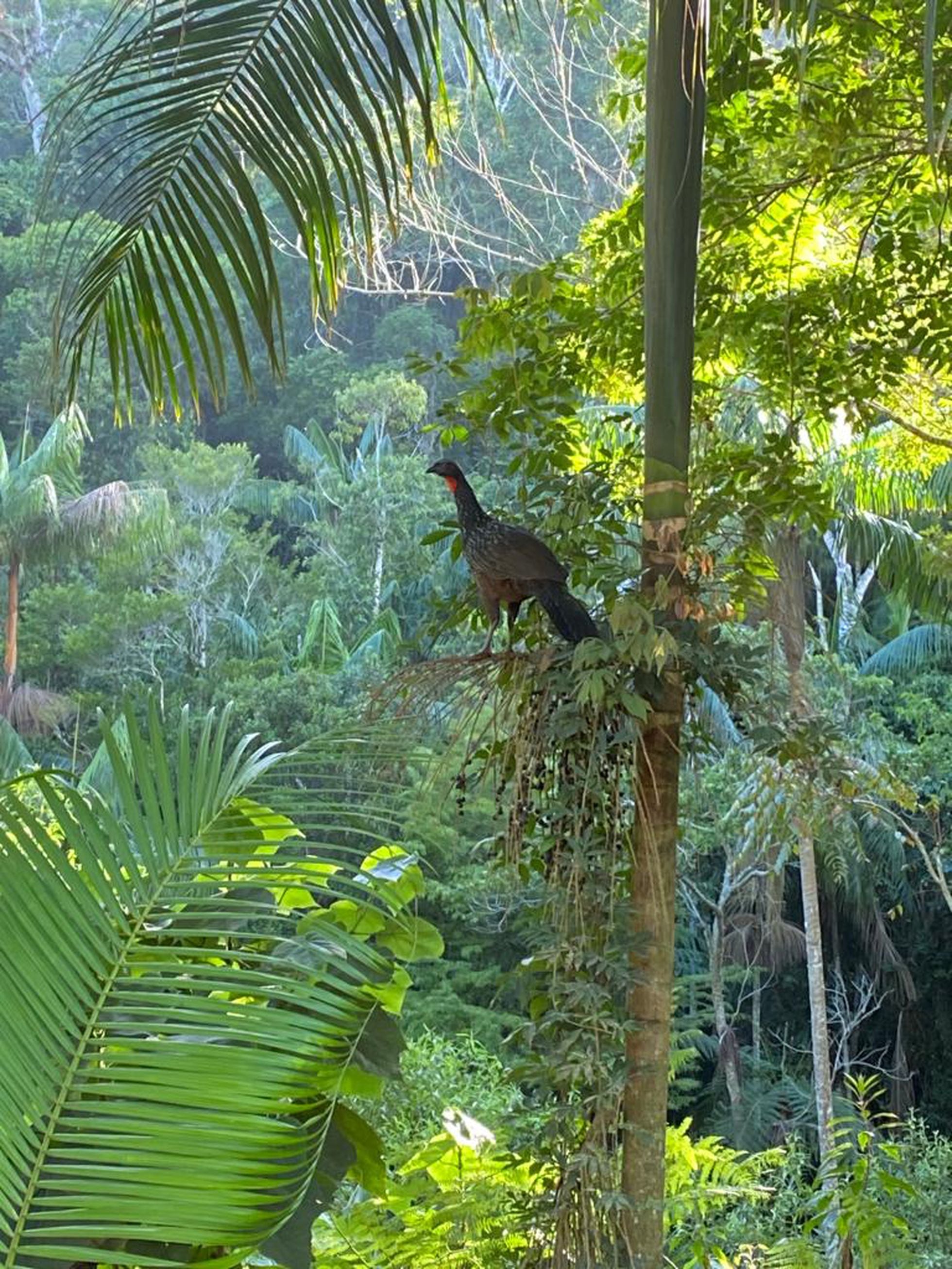This image captures a vibrant, dense jungle scene brimming with lush greenery and towering trees. A central feature is a tall, slender tree on the right side, characterized by a greenish-brown trunk and thin branches. Among its branches, dry leaves provide a perch for a striking bird. The bird, resembling a peacock, is predominantly black with a contrasting gray underside, and an unmistakable splash of orange-red on its neck. The bird, seen in a side view, faces left and stands on the tree bark, showcasing its slender black beak. Thick tropical foliage, with large palm-like leaves, dominates both the upper left and bottom right corners of the image, suggesting a dense and vibrant jungle canopy. Sunlight filters through the leaves, highlighting sections of the scene and casting dappled light patterns throughout the composition. The background reveals numerous similar trees with thin trunks, reinforcing the image’s lush, tropical atmosphere.